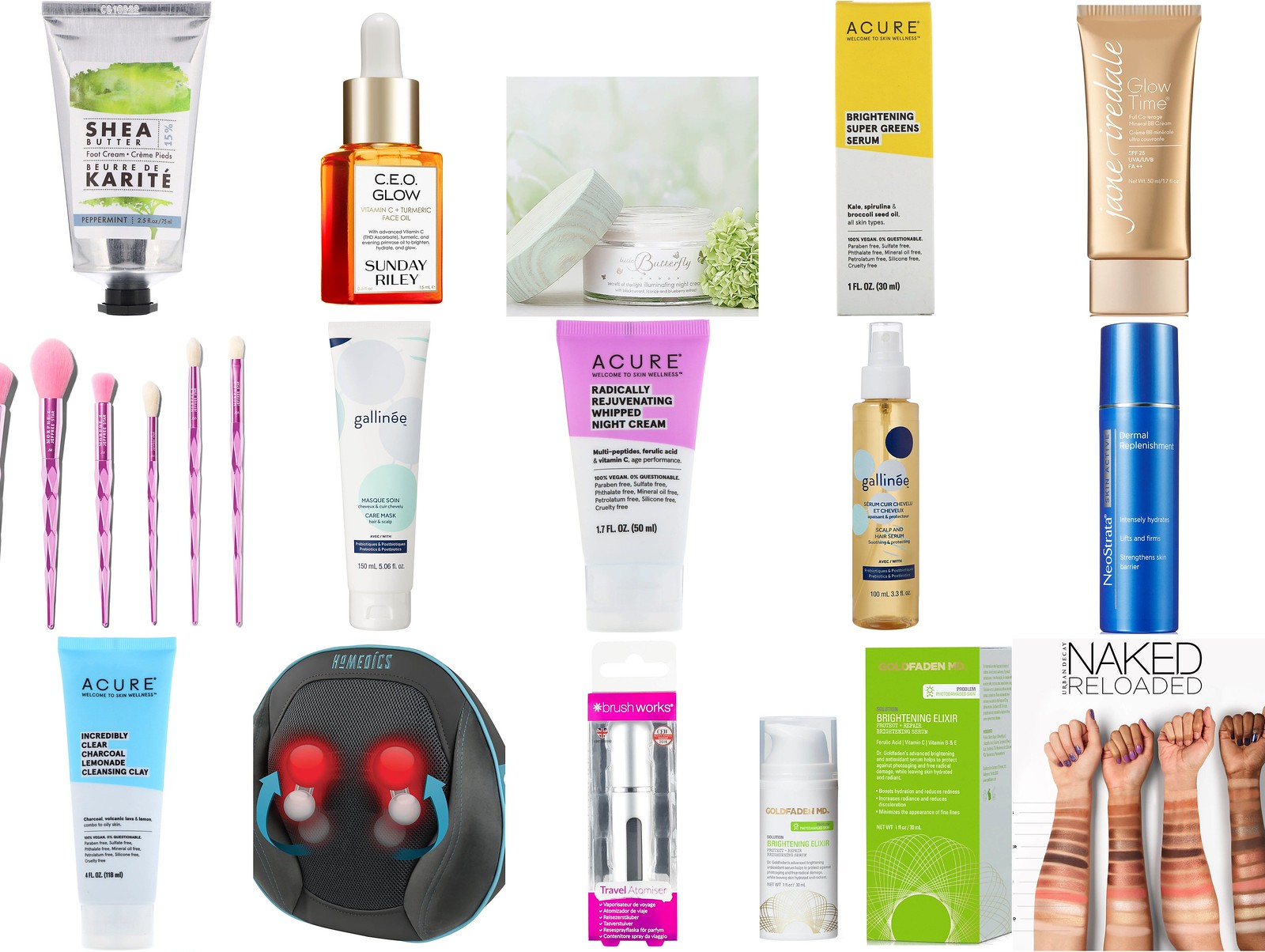This promotional image showcases a diverse array of 15 beauty products arranged neatly in three rows on a webpage. Each row contains five items, highlighting various brands and types of beauty essentials.

In the top row, you'll find a range of products, starting with "Shea Carite" in a sleek white bottle adorned with green labeling. Following this, you'll see "C.E.O. Glow" by Sunday Riley, distinguishable by its clear bottle filled with vibrant orange liquid. The row also includes a product labeled "Acure."

The middle row continues to showcase a mix of beauty items, featuring another "Acure" product in a light blue bottle. 

In the bottom row, there's a striking box labeled "Naked Reloaded" positioned in the lower right corner. The box design is particularly eye-catching, decorated with images of four arms and hands displaying smears of different makeup products. Additionally, there is an "Acure" product in a yellow and white box.

Centrally located to the left, a bundle of makeup brushes with elegant pink handles adds a touch of sophistication to the collection. 

This comprehensive display effectively presents a variety of skincare and makeup products, illustrating the wide selection available for beauty enthusiasts.